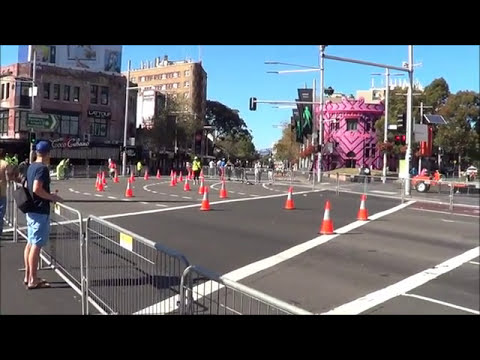Situated in a bustling downtown area, this photograph captures a city street transformed for a marathon event. Numerous orange traffic cones line the road, effectively creating lanes for runners. Metal temporary fencing borders the race route, with spectators gathered behind, eagerly watching the participants. A prominent pink building, resembling a castle, stands on a street corner in the distance, adding a splash of color to the urban backdrop. One noticeable runner, clad in yellow, heads towards the onlookers during this daytime event. The sky overhead is clear and blue, emphasizing the vibrancy of the cityscape around the closed-off street. Parked vehicles, street signs, and lamps are visible, enriching the detailed city environment. The scene also features a man in shorts, a t-shirt, and a hat, positioned behind the guardrail, observing the ongoing race.